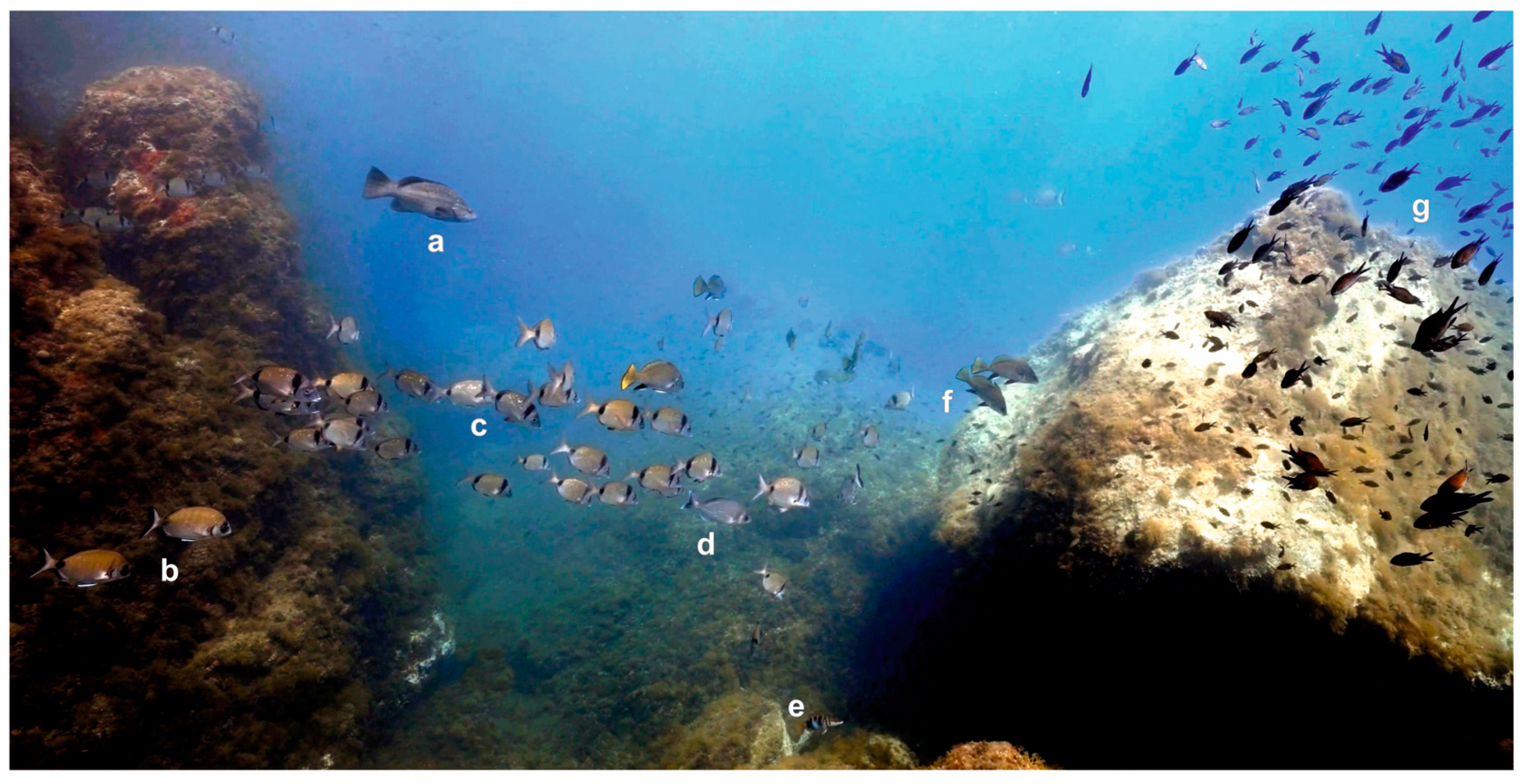This horizontally aligned rectangular underwater photograph features a variety of marine life and structures. Dominating the right side from the bottom to the middle is a large, white or light gray rock covered with brownish-green algae, suggesting a well-established ecosystem. To the left, a darker brown coral reef contrasts sharply with the white rock. In the upper right corner, a vibrant school of tiny blue fish adds a burst of color, while the middle-left area displays slightly larger fish with brown and white markings. The bottom of the picture reveals additional rock formations and seaweed, contributing to the photo's rich texture.

Further enriching this scene, the central area features the deep blue waters of the ocean, which lightens towards the top. The background consists of varying hues of blue and green, enhancing the aquatic depth. Interestingly, each fish species in the photo is marked with small white letters ranging from A to G, starting from the left side and spreading across to the right, making it an educational as well as a beautiful display of underwater life.